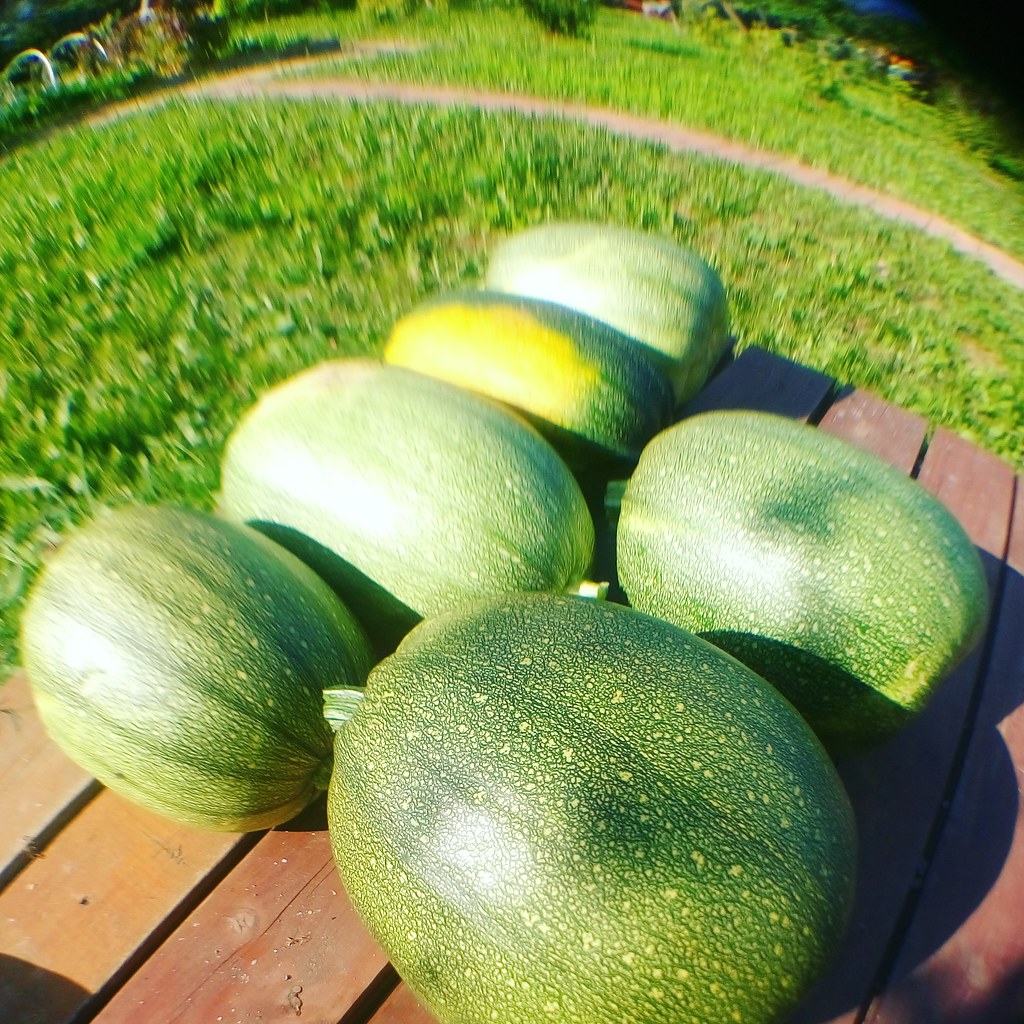The image features a diagonal view of a redwood-colored picnic table with wide slats, showcasing six fruits or vegetables, possibly a type of green squash or melon. These are arranged in two rows: one row of four and one row of two. The produce exhibits varying shades of green with light green backgrounds and dark green squiggle patterns, and one of them near the top center has a distinct yellow patch. The scene is bathed in sunlight, with reflections and shadows indicating the sun is coming from the left side. The background consists of vibrant green grass, a small trail, and a garden area hinting at where the produce may have been grown. This background is somewhat out of focus and appears slightly curved, suggesting the photograph was taken with a fisheye or wide-angle lens, giving it a radial blur effect. The overall setting is outdoors on a bright, sunny day.